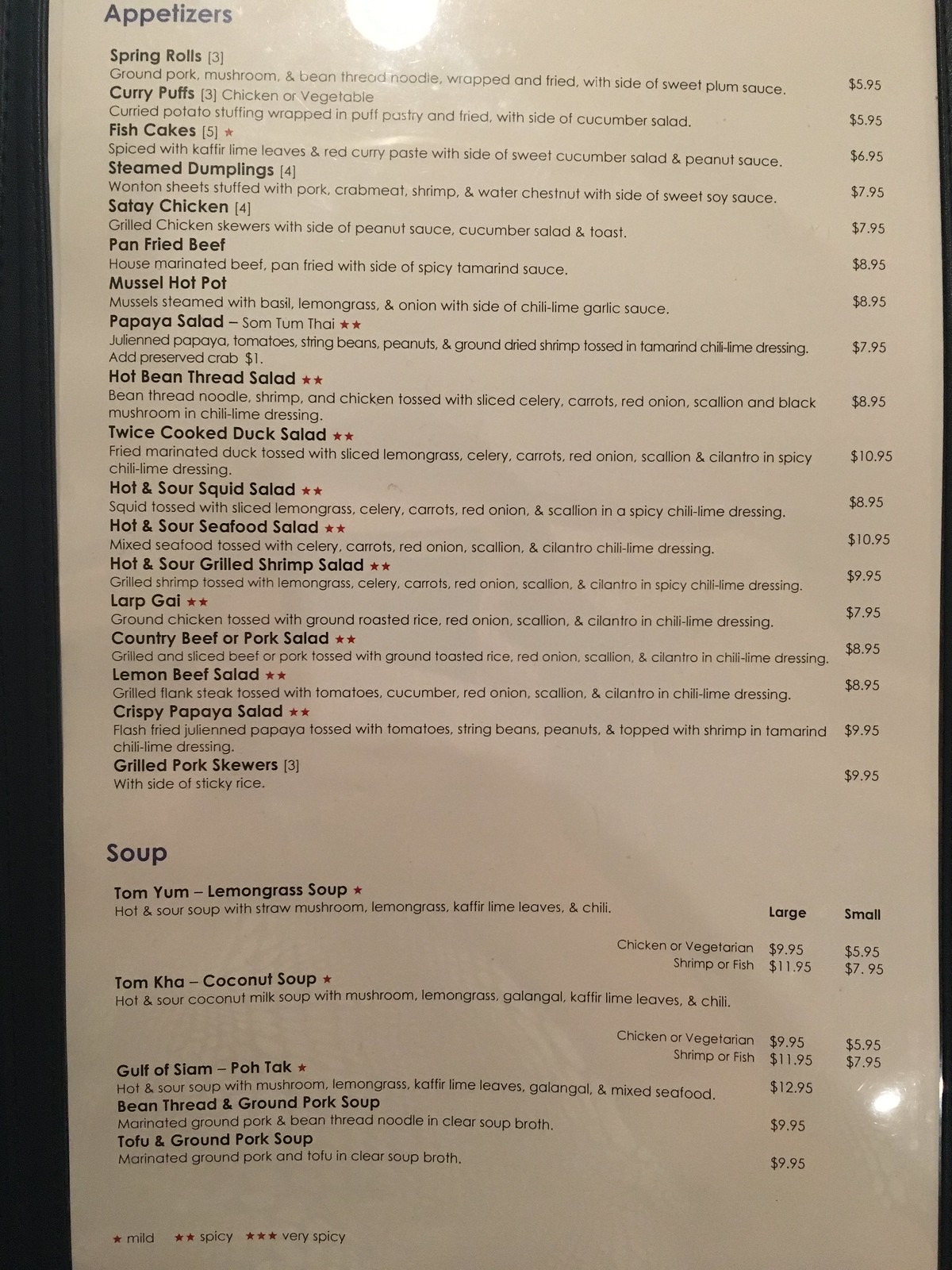This image displays a restaurant menu with an elegant white background and black text. The menu is divided into sections, with the top left corner dedicated to "Appetizers". The appetizer titles include an array of tempting options: Spring Rolls, Curry Puffs, Fish Cakes, Steamed Dumplings, Satay Chicken, Pan-Fried Beef, Mussel Hot Pot, Papaya Salad, Hot Bean Thread Salad, Twice Cooked Duck Salad, Hot and Sour Squid Salad, Hot and Sour Seafood Salad, Hot and Sour Grilled Shrimp Salad, Barbeque Guy, Country Beef or Pork Salad, Lemon Beef Salad, Crispy Papaya Salad, and Grilled Pork Skewers. 

Below the appetizer list, the "Soup" section features: Tom Yum Lemongrass Soup, Tom Kha Coconut Soup, Gulf of Siam Potak, Bean Thread and Ground Pork Soup, and Tofu and Ground Pork Soup.

Additionally, the menu includes a spiciness guide at the bottom, indicating the level of heat for each dish. One red star represents mild spice, two red stars indicate spicy, and three red stars signify very spicy. Notably, none of the items listed on this menu are marked as very spicy. Most of the salads from Papaya Salad to Crispy Papaya Salad are marked with two red stars, denoting a spicy flavor, while Fish Cakes are marked with one red star, indicating a mild spice level.

The detailed layout and clear categorization make it easy to understand the offerings and spice levels, enhancing the dining experience.